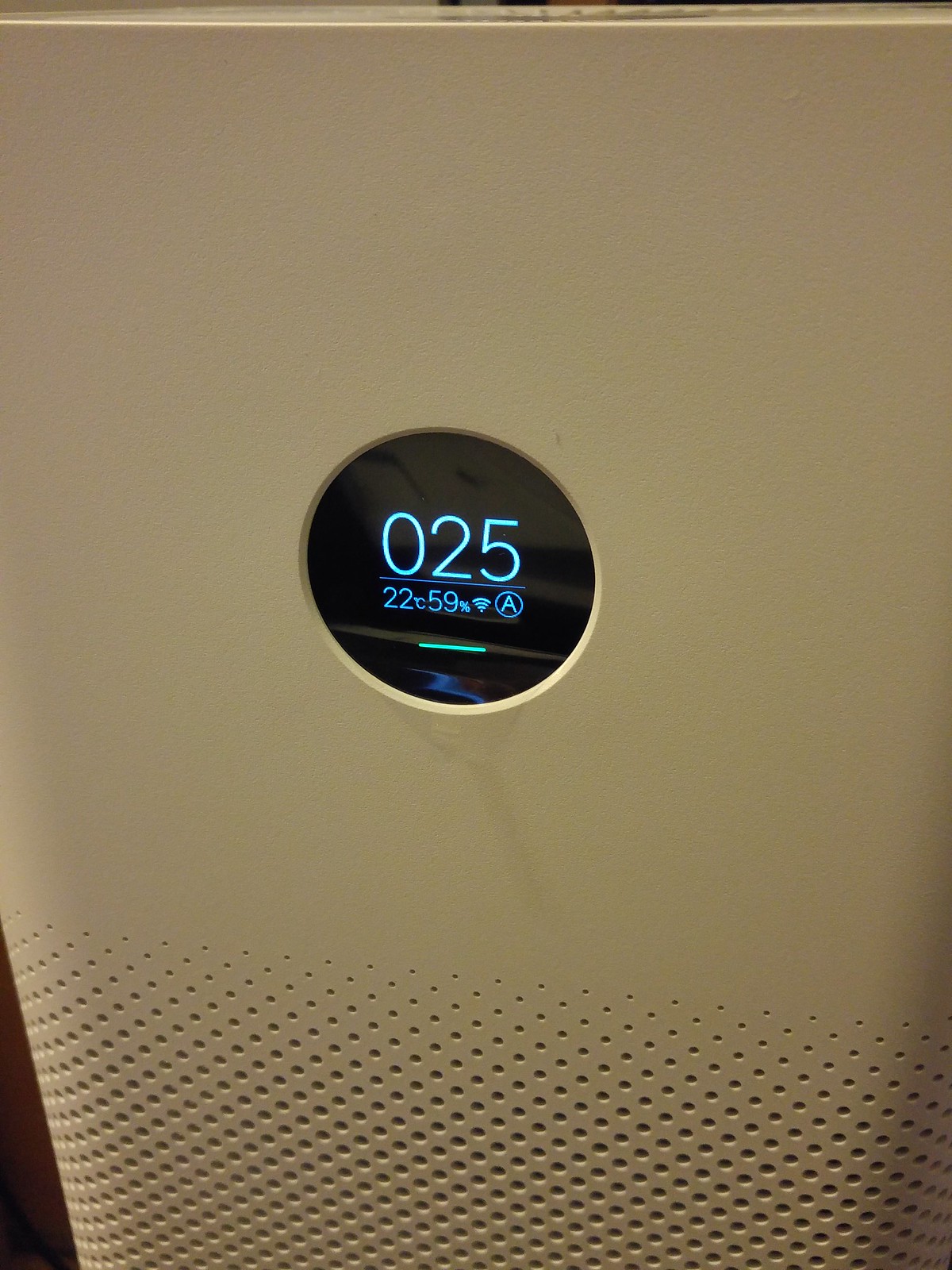This photograph showcases a sleek, modern appliance in an off-white color. At the bottom, a ventilation grille with small circular cutouts arranged in a diamond pattern adds a functional and aesthetic detail. Centrally located on the appliance is a black, circular LED display screen. The screen prominently displays the numbers "025" at the top, with "2259" underneath. Alongside these numbers, a Wi-Fi symbol and a letter "A" enclosed in a circle are also visible. The design is minimalist, with no additional buttons or features visible on the front of the appliance, emphasizing its clean and contemporary appearance.